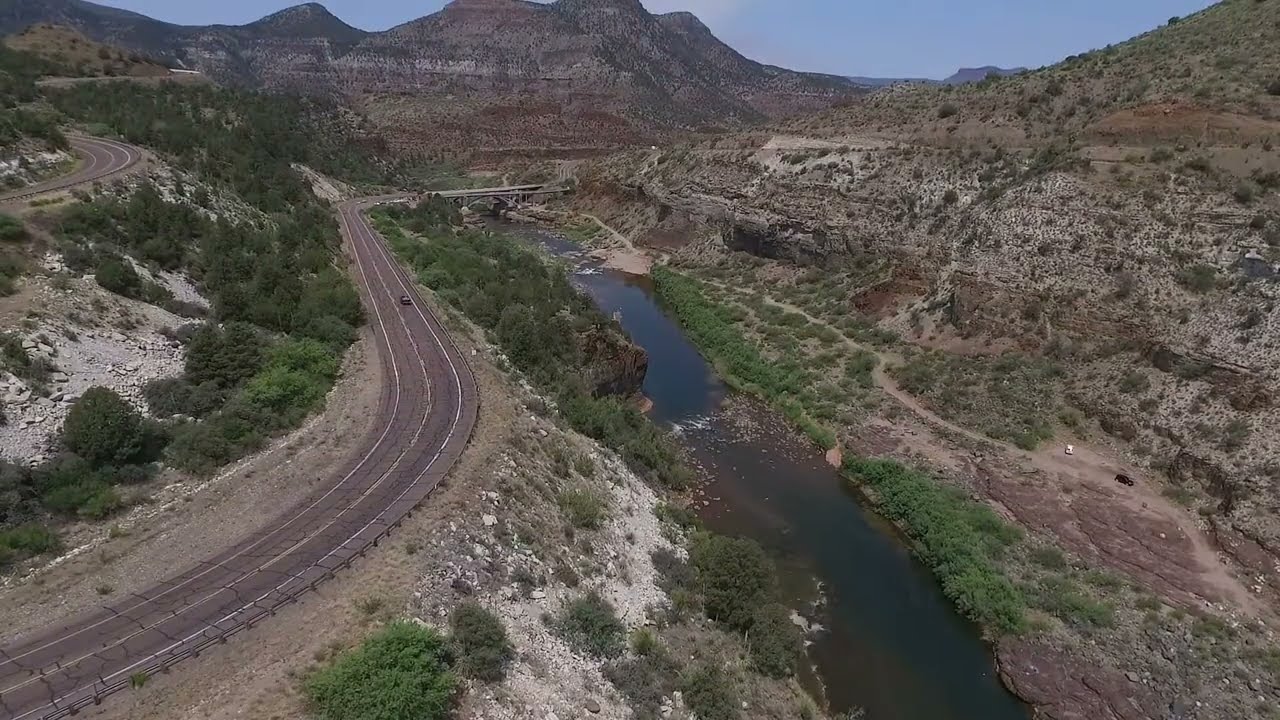An aerial photograph captures a vast, rugged landscape characterized by a rocky mountain range with sloping roads and a serene valley cutting through the center. The terrain is interspersed with patches of green trees and bushes among the dominant brown hues of the rocks and rubble, typical of a semi-arid, canyon-like environment. A winding highway meanders through the left side of the image, snaking up and around the mountains, and features a single vehicle, highlighting the road’s desolation. The waterbody, likely a river or stream, cascades through the valley, flowing cleanly albeit slightly murky, flanked by a path that invites hikers to explore the scenic views. The sky above is a clear blue, and a big mountain stands prominently in the background, underlining the peaceful yet imposing beauty of the natural setting.